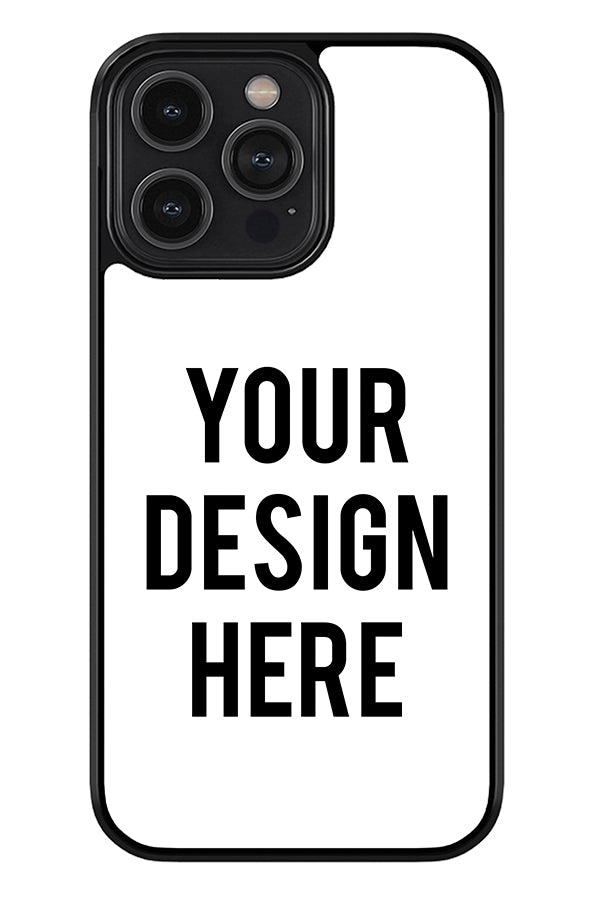The image is an advertisement for creating custom phone cases. It displays the back of a recent iPhone model, likely an iPhone 13 or 14 Pro, characterized by its three camera lenses arranged in a square at the top-left corner. The phone case features a black outline with a white interior, and large, bold, black text that reads "Your Design Here" across the center. The phone's back has some additional, smaller circular cutouts, possibly for a light meter and a microphone. The background of the image has been photoshopped out to emphasize the phone case. The overall effect is a minimalist template, inviting users to upload their own design, which the company will print and send, resulting in a unique and personalized phone case.